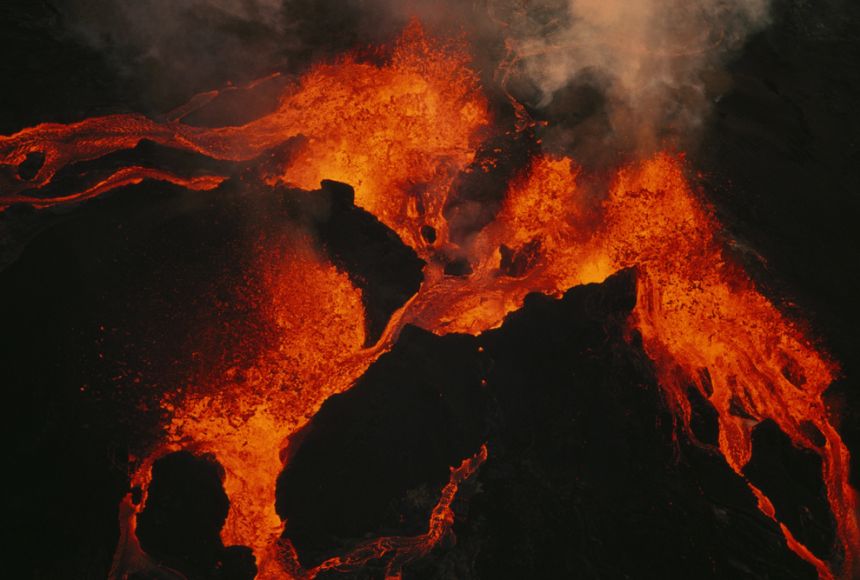The image captures an intense close-up of an active volcano amidst a dynamic eruption. The volcano’s silhouette is a deep, pitch-black, contrasting starkly against the vibrant, chaotic lava flows. Streams of molten lava, in vivid shades of orange, red, and yellow, burst dramatically from the summit and snake their way down the slopes, spilling towards the lower right, left, and center of the frame. The top portion is shrouded in thick, billowing gray smoke, adding to the sense of raw power and intensity. The scene is enveloped in darkness, giving no indication of day or night, and the incandescent lava barely illuminates its surroundings, emphasizing the profound gloom. The overall sharpness of the photograph allows these details to stand out crisply against the void, making the image a striking depiction of nature’s unstoppable force.